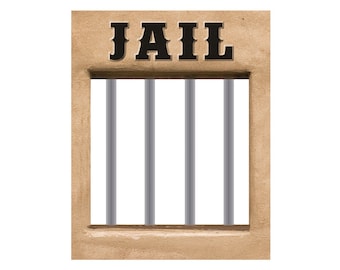The image depicts a light brown, slightly shiny wooden square set against a plain white background, giving it a clean, minimalist appearance. At the center of the wooden square, there's a smaller, white square with four vertical, steel-gray bars, resembling a jail cell window. The word "JAIL" is prominently displayed in bold, black letters at the top of the wooden square. The overall composition gives the impression of a simplified, emoji-like representation of a jail cell.